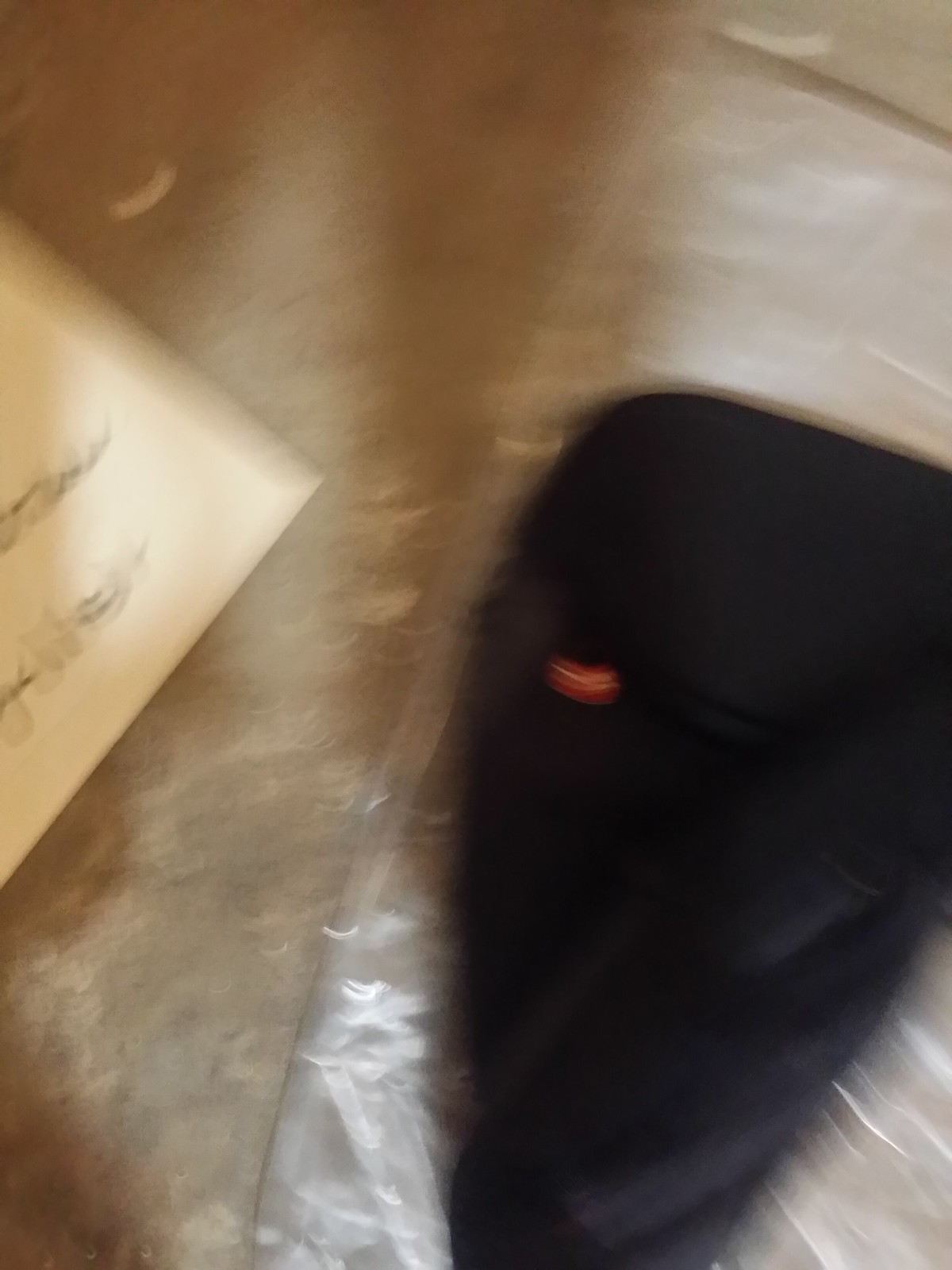A heavily blurred, low-light photograph shows a scene with difficult-to-discern details due to significant motion upon capture. On the right side of the image, there is a black, fabric-like object with a small red dash, possibly a logo. To the left, there appears to be a handwritten note on a piece of paper, though the text is indecipherable. The photo has a plastic background and is taken in a rectangular frame.